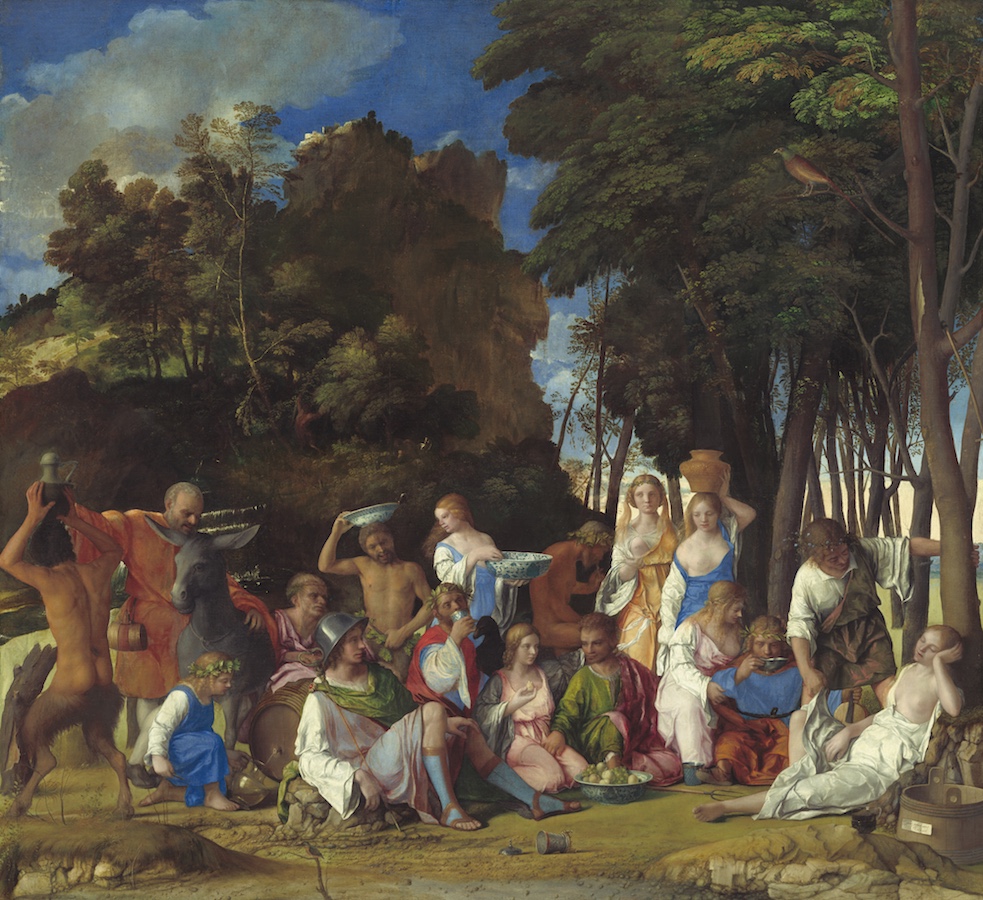This oil painting captures a vivid medieval scene by a serene pond, where a gathering of approximately twenty people, dressed in period attire reminiscent of Roman times, are spread out on a lush grassy area surrounded by trees. The background features a bright blue sky with meticulously painted clouds, along with a distant butte crowned with trees. Central to the composition is a large ceramic bowl brimming with apples, around which people are seated. 

Numerous women in the scene are partially clad, with their dresses hanging off and breasts exposed, engaging in various activities. Notably, one woman in the middle holds a striking blue ceramic bowl with a blue floral design, while another balances a terracotta pot on her head towards the back. There are also a few men dressed in overalls, long socks, and sandals, evocative of old Roman days, with one shirtless man carrying a bowl on his head.

Adding to the fantastical element, a half-human, half-horse figure, viewed from behind, stands on the left side, holding a water container above his animal-like legs. This centaur-like character, alongside the others, contributes to the mythic and otherworldly ambiance of the scene. Scattered across the scene are various containers—vases for water, jugs, and pitchers—indicating the act of drawing and storing water.

The painting beautifully combines elements of mythology, medieval culture, and detailed human interactions, offering a richly detailed tableau that invites viewers into its historical and fantastical world.